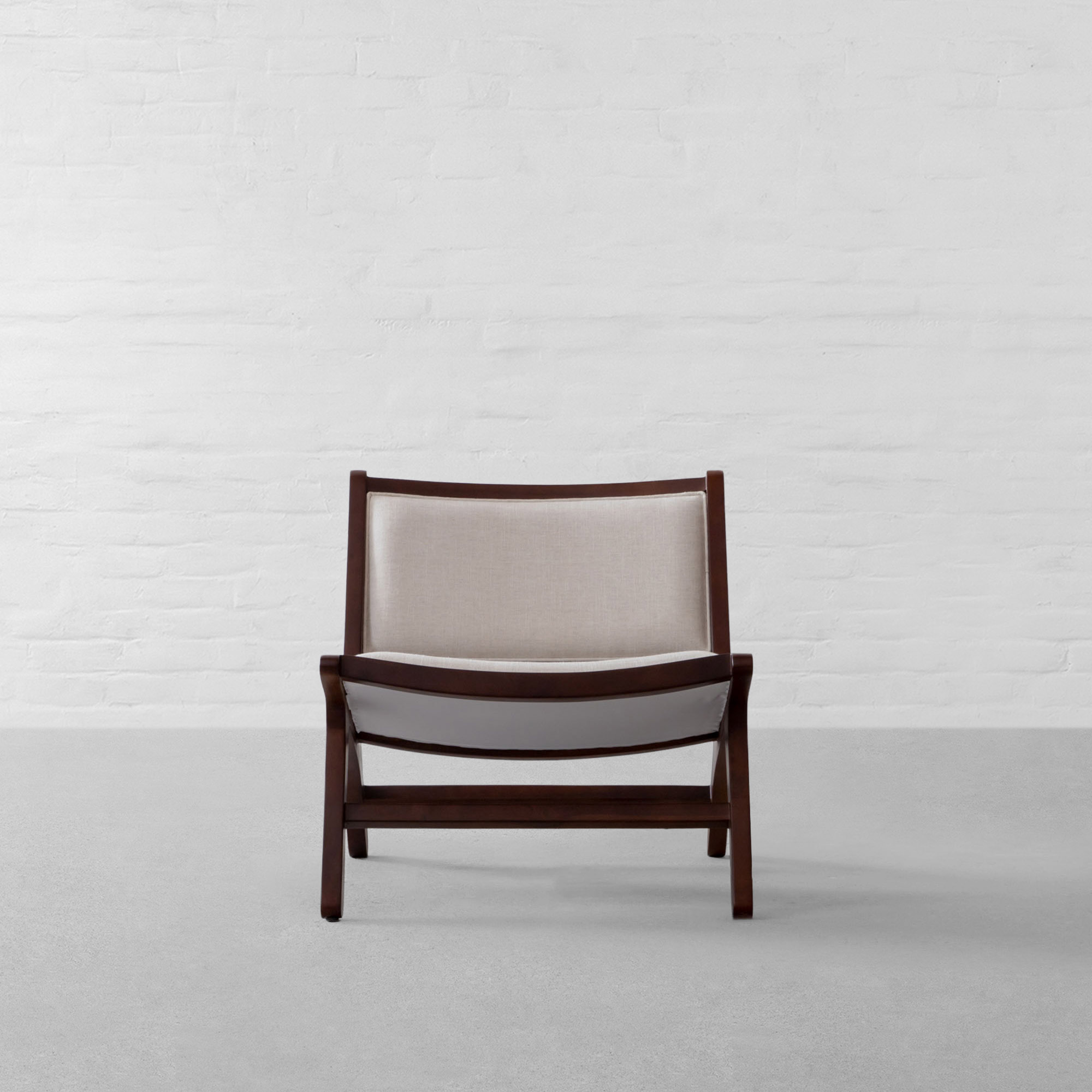In this computer-generated, lifelike photograph, a singular, old-style fashioned folding chair is prominently featured. The chair has a sturdy, dark brown wooden frame with four legs and two support beams across the bottom. The seat and back cushions are upholstered in a light gray fabric, creating a stark contrast against the darker wooden elements. The image captures the chair in a mostly featureless room, where it sits on a solid light gray carpet that matches the cushions. Behind the chair, a white painted wall reveals the subtle indents of the underlying bricks, adding a touch of texture to the otherwise plain space. The photograph is square-shaped and meticulously detailed, showcasing a realistic shadow cast by the chair onto the floor. The angle of the shot makes the chair appear almost partially folded, although it is not, creating a captivating illusion of depth and dimension.